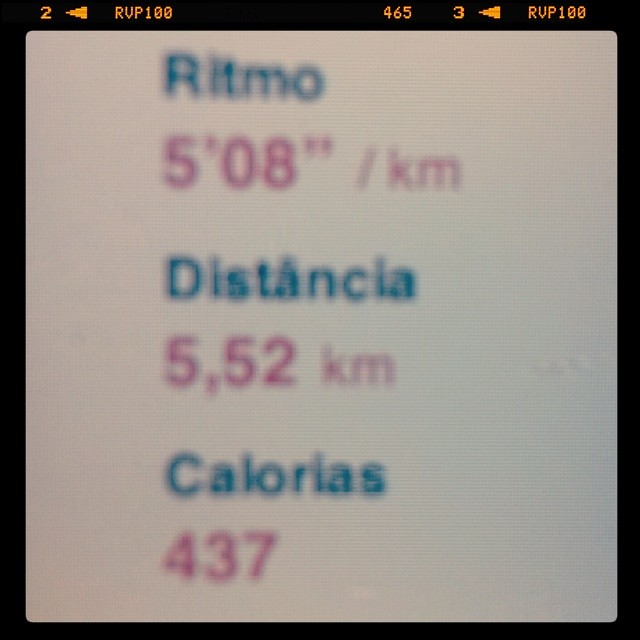This image features a black, square-shaped border with a white-background sign in the middle, though it is slightly out of focus and blurry. Along the top edge of the black border, there is orange digital text showing a sequence of numbers and letters: it starts with "2" followed by a left-pointing triangle and "RVP 100," then "465," and finally "3" followed by another left-pointing triangle and "RVP 100." 

Inside the white center of the square are three lines of text, each in different colors. The first line at the top reads "RITMO" in blue, followed by "5 feet 0.8 inches / KM" in red. The second line says "DISTANCIA" in blue, with the numbers "5.52 KM" in red directly below it. The third line reads "CALORIAS" in blue, accompanied by the number "437" in red. The details are presented in Spanish, likely indicating rhythm (RITMO), distance (DISTANCIA), and calories (CALORIAS). The overall composition of the image, despite its blurriness, suggests a digital display of some measured quantities, possibly related to fitness or exercise metrics.